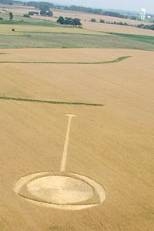The semi-aerial, overhead image showcases expansive farmland, predominantly featuring a brown-colored wheat or corn field with patches of greener grass interspersed. Dominating the brown field is an intricate crop circle pattern resembling a paddle or shovel, characterized by a long handle and an oval shape at its base. Nested within this oval are concentric shapes: a half-circle and a smaller full circle, each distinct in color. Above the shovel-like form, two elongated patterns are etched into the field: one shaped like a hockey stick and the other a straight line. The landscape extends towards a verdant horizon scattered with trees, including evergreen varieties, merging into a distant skyline. The contrast between the yellowish-brown crops and the vibrant green patches enhances the visual complexity of the scene.